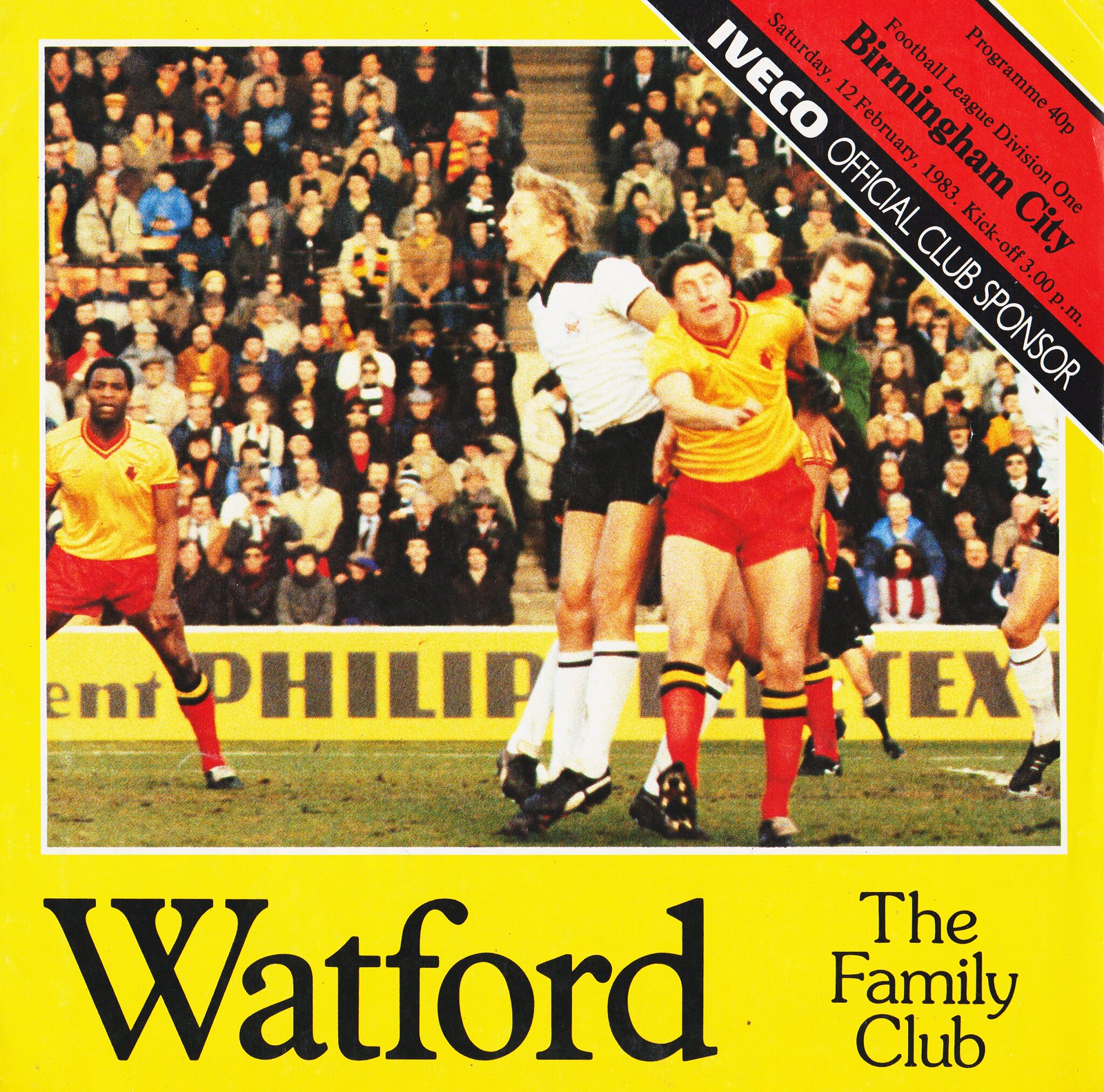The image is a square, vintage cover of a soccer program from 1983. The thick yellow border, more pronounced at the bottom, frames a central photograph capturing a live soccer match. This vibrant photo features two teams: one in yellow and red jerseys, matching the yellow border, and the other in white and black jerseys. A young man in the white and black jersey is depicted mid-jump, likely aiming to head the ball, while being nudged by an opposing player in a yellow and red jersey. 

Above the main photograph, a red text banner in the upper left corner reads "Program 40 Pence, Football League Division I, Birmingham City, Saturday, 12 February 1983, kickoff at 3 p.m.," underscoring the program's historical context. The image also shows a crowd of spectators in the stands, enhancing the dynamic atmosphere of a professional soccer match. The bottom of the cover prominently displays the title, "Watford Family Club," highlighting the program’s association with the Watford soccer team. Additionally, it mentions the official club sponsor, Iveco. The overall aged appearance, including some yellowing and blemishes, adds to its nostalgic charm.